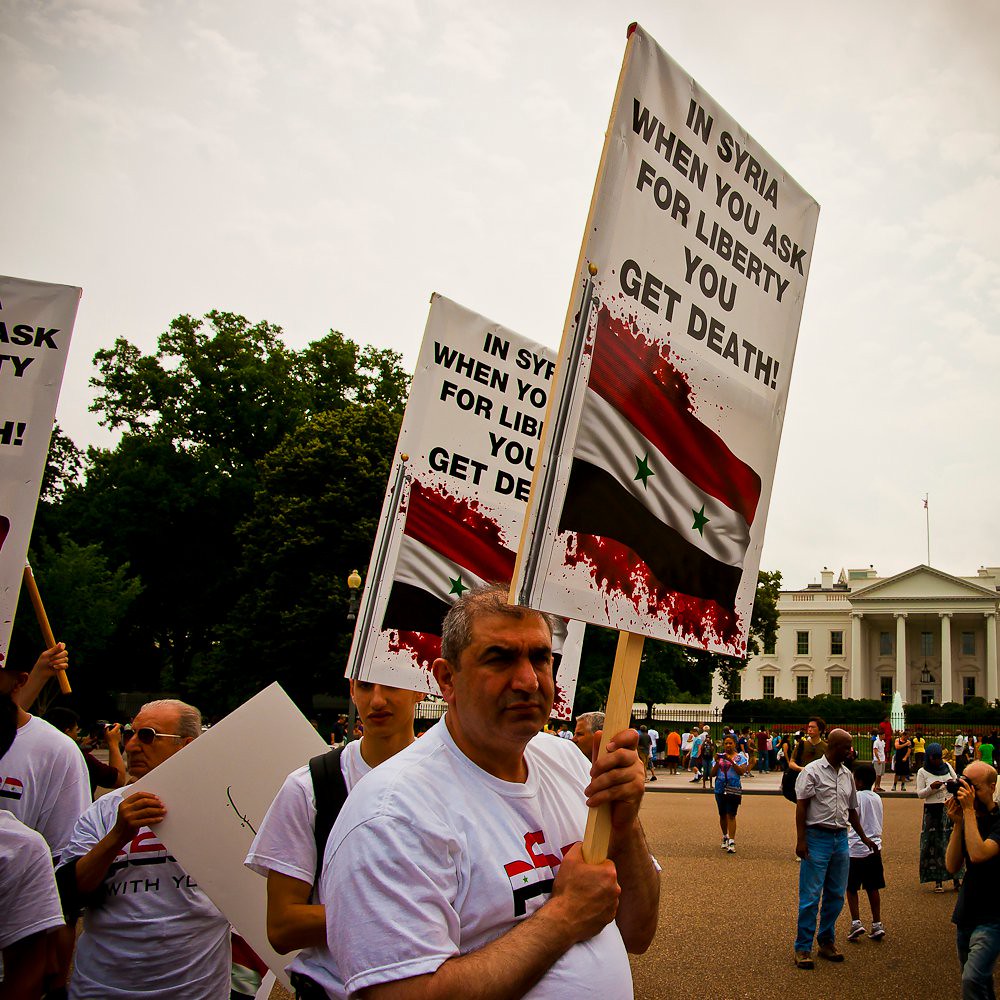The color photograph, taken in a square format, captures a detailed scene of a protest occurring on outdoor grounds, believed to be in front of the White House. The ground is covered with brown soil and populated with numerous individuals. Central to the image is a group of protesters, all donned in white shirts featuring a flag on the chest. They hold up white placards bearing the message, "In Syria, when you ask for liberty, you get death," accompanied by an illustration of the Syrian flag stained with red splatters resembling blood. The focal point is a man standing prominently at the center bottom, facing the viewer and holding up the sign, with another person partially visible behind him carrying the same message. Other protesters with identical signs are dispersed throughout, while some bystanders are seen taking photos. In the background, a tree and a white building, presumably the White House, are visible, framed under a sky with scattered white clouds. The photograph is a vivid depiction of the protest, rendered in a realistic, representational style.